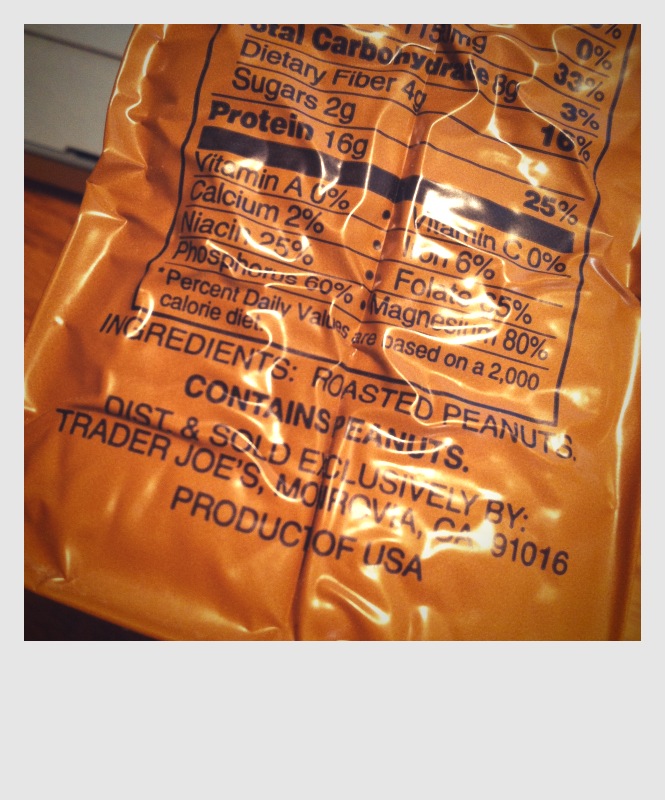This meticulously detailed image showcases the nutritional and ingredients labels on a vacuum-sealed bag of roasted peanuts, which comes in a vibrant orange packaging. The sole ingredient listed is roasted peanuts, confirming it contains peanuts and is a product distributed and sold exclusively by Trader Joe's, located in Monrovia, California, with the ZIP code 91016. As a product of the USA, the label highlights its nutritional values: containing 16 grams of protein, 2 grams of sugar, 4 grams of dietary fiber, and a total of 8 grams of carbohydrates. The label also specifies the presence of key nutrients, reflecting 0% Vitamin A, 2% Calcium, 25% Niacin, 60% Phosphorus, 0% Vitamin C, 6% Iron, 35% Folate, and 80% Magnesium.